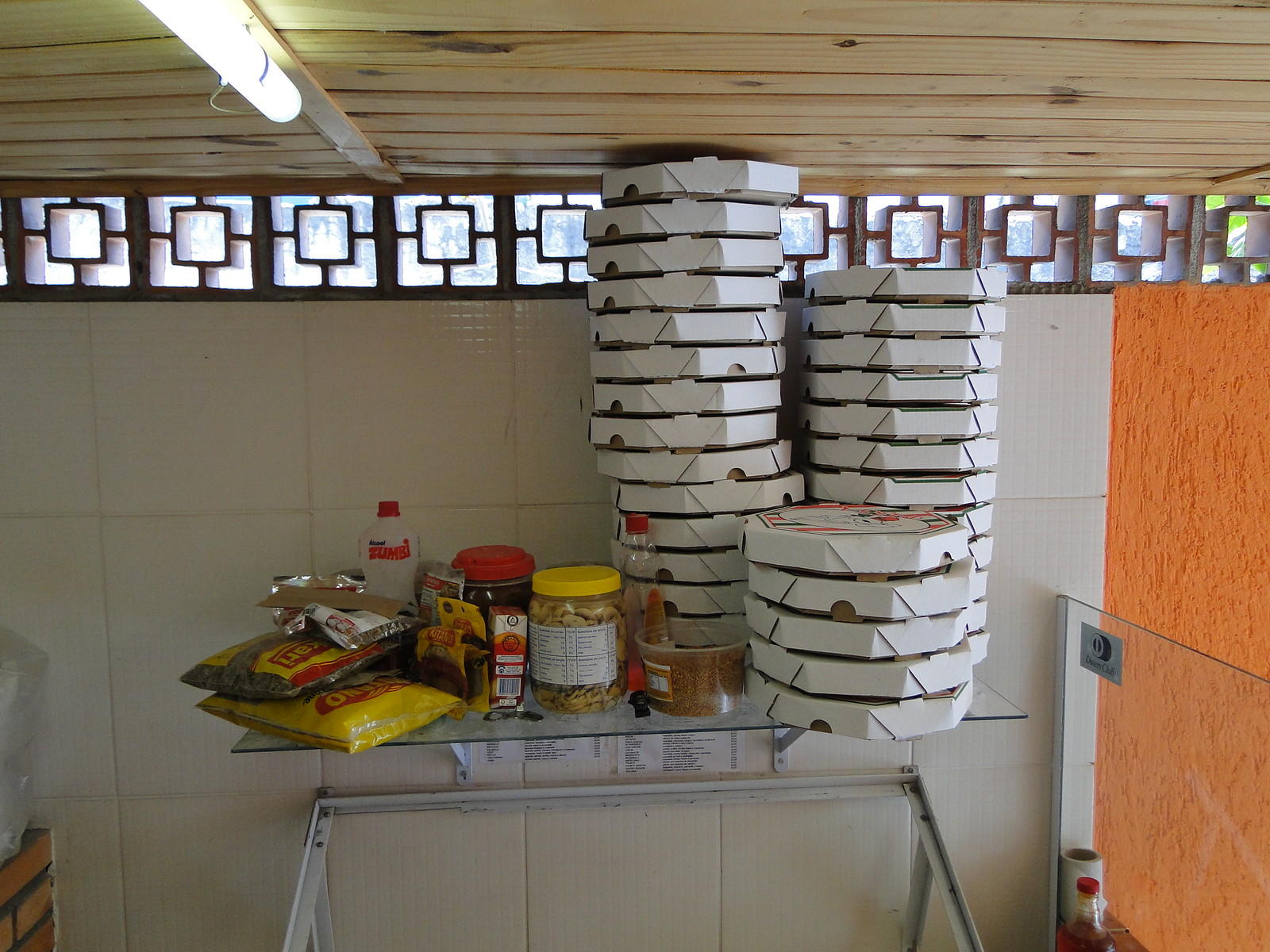The image depicts a bright room with white tile walls, featuring an arrangement of stacked round boxes, resembling pizza boxes, on a glass countertop that's positioned against the wall. There are three distinct stacks of these boxes: one towering with approximately 14 boxes, another with around 12, and a smaller stack with 5 boxes. The tabletop also holds various jars filled with different foods, packs of ingredients, seasonings, and a menu at the bottom. Light wood paneling with an attached light fixture adorns the ceiling, which enhances the daytime ambiance visible through small decorative windows. The room's background reveals an intriguing mix of white tiles, brickwork between windows, and an orange wall separated by a glass divider.